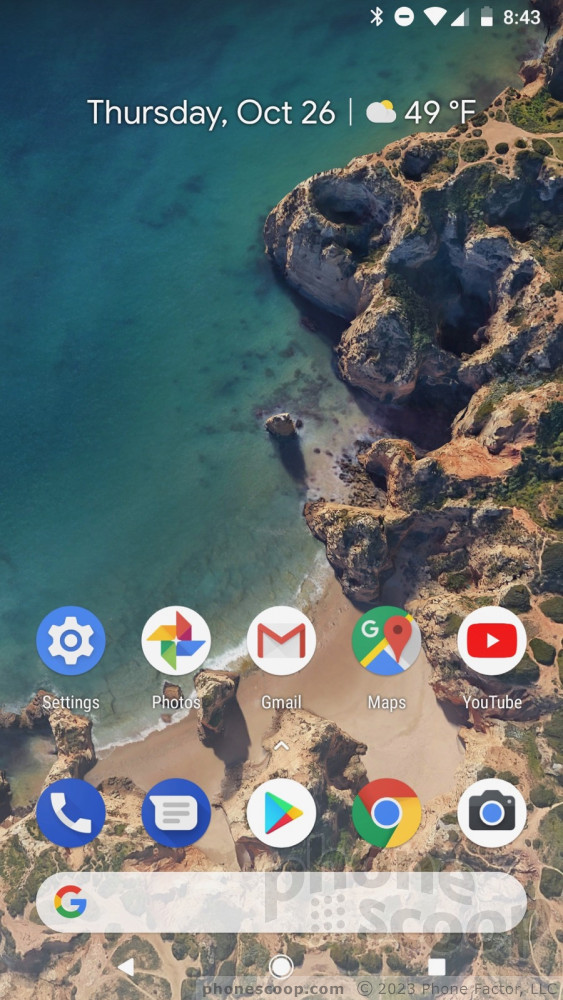The image displays a phone screen with several details. At the top of the screen, the status bar shows Bluetooth connectivity, a circle with a line through it, signal bars for cellular and Wi-Fi connections, and a half-full battery icon. The time is 8:43, and the date is Tuesday, October 26th. The weather is indicated as 49 degrees Fahrenheit and mostly cloudy.

The wallpaper features an aerial view of a coastline with turquoise blue ocean waves meeting the shore. The sandy beach and cliff are also visible in the image.

At the bottom of the screen, various app icons are aligned, including Settings, Photos, Gmail, Maps, YouTube, Phone, Text Messages, Google Play, Google Search, and Camera. A Google search bar is situated right above these icons. 

Additionally, there's a watermark on the bottom right corner that reads "PhoneScoop" in a stylized format and the website "PhoneScoop.com" is displayed just below the navigation buttons (Back, Home/ Circle, and Square).

The colors present in the image include shades of brown, turquoise blue, red, white, green, blue, orange, and yellow.